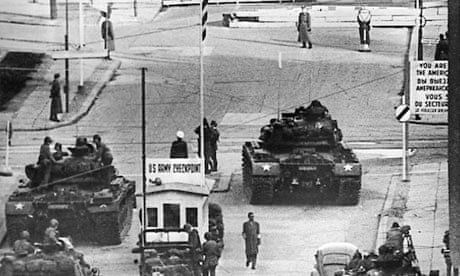This detailed black-and-white photograph, likely from the 1960s or 70s, depicts a bustling scene at a U.S. Army checkpoint, possibly during wartime. The image appears to be taken from an elevated vantage point, possibly from a building or hillside. Dominating the scene are two large tanks marked with stars, each carrying several soldiers in full uniform who might be holding weapons. Various military vehicles, including trucks and a notable Volkswagen Beetle, are scattered throughout the area. Civilians and soldiers intermingle, some walking or standing around, while others sit atop the tanks. The checkpoint features a small white building with a sign that reads "U.S. Army Checkpoint," and another partially legible sign suggests it might be an emergency area. The presence of long-coated military personnel hints at a historical setting, potentially during World War II. The general environment, with people going about their day amidst the military activity, coupled with the language on the signs, raises the possibility that this scene could be somewhere in Europe, perhaps even France.